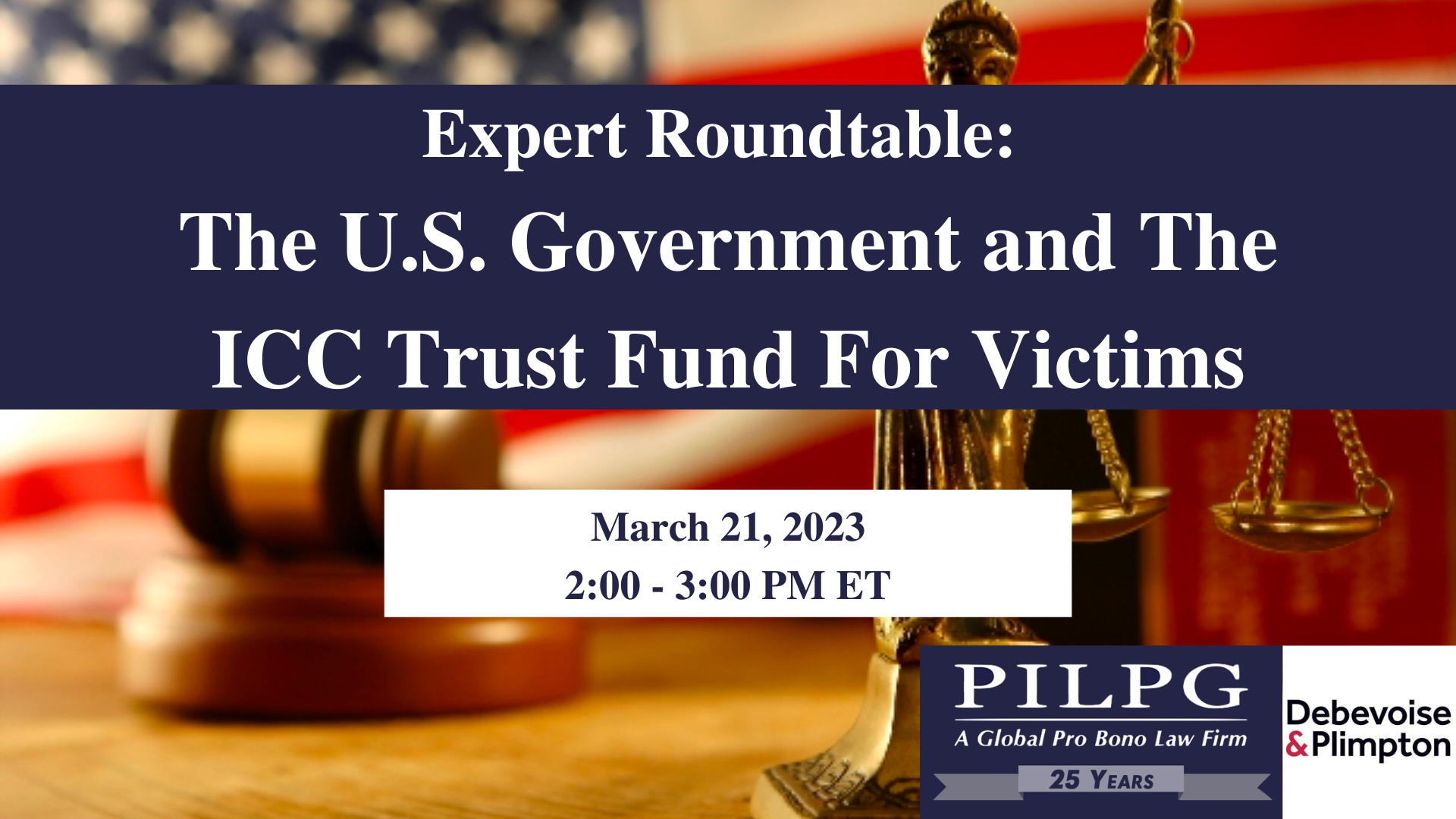The advertisement showcases an upcoming event against a backdrop featuring a blurred American flag and a wooden desk with a gavel, symbolizing justice. Prominently in focus is a bronze statue of Lady Justice holding scales. Across the image's top portion is a dark blue banner with white text that reads "Expert Roundtable: the US Government and the ICC Trust Fund for Victims." Below this banner, within a white text box, the event date and time are detailed: "March 21st, 2023, 2–3 p.m. ET." In the bottom right corner, a blue text box states "PILPG, a global pro bono law firm, 25 years," and adjacent to it, on a white background, is the name "Debevoise & Plimpton." This detailed image is likely an announcement slide for a significant legal roundtable event.